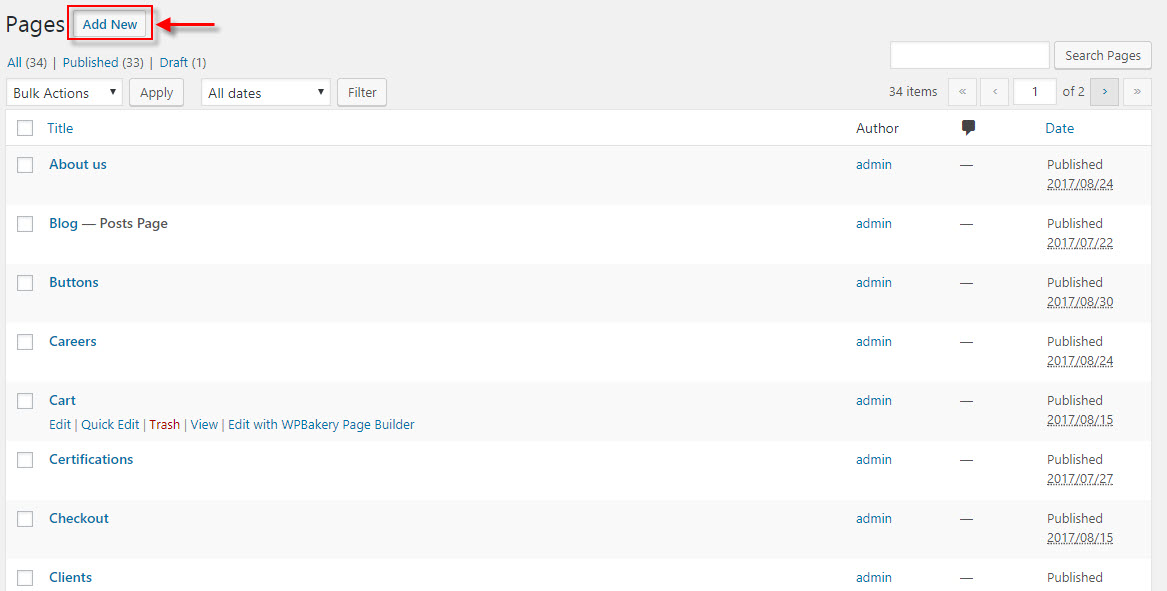The image depicts a digital interface for managing website content, likely a content management system (CMS) designed for organizing articles, posts, and various written materials. The interface appears on a computer monitor screen and features a toolbar at the top. In the top left corner, the word "Pages" is prominently displayed. To its right, a button labeled "Add New" is highlighted with a red box and an inward-pointing red arrow from the right side, suggesting it is part of a tutorial indicating where to click to add new content.

Below this toolbar are several tabs and options, including "All" with a count of 34, "Published" with 33, and "Drafts" with one entry. A search bar allows users to search through the pages, and a dropdown menu labeled "Bulk Actions" offers options for batch processing. There are additional options to filter content by date. The interface lists various page titles such as "About Us," "Blog," "Buttons," "Careers," "Cart," "Certifications," "Checkout," and "Clients," indicating diverse categories that are being managed.

The structured layout and detailed options suggest this is a robust system intended for organizing and managing website content efficiently.